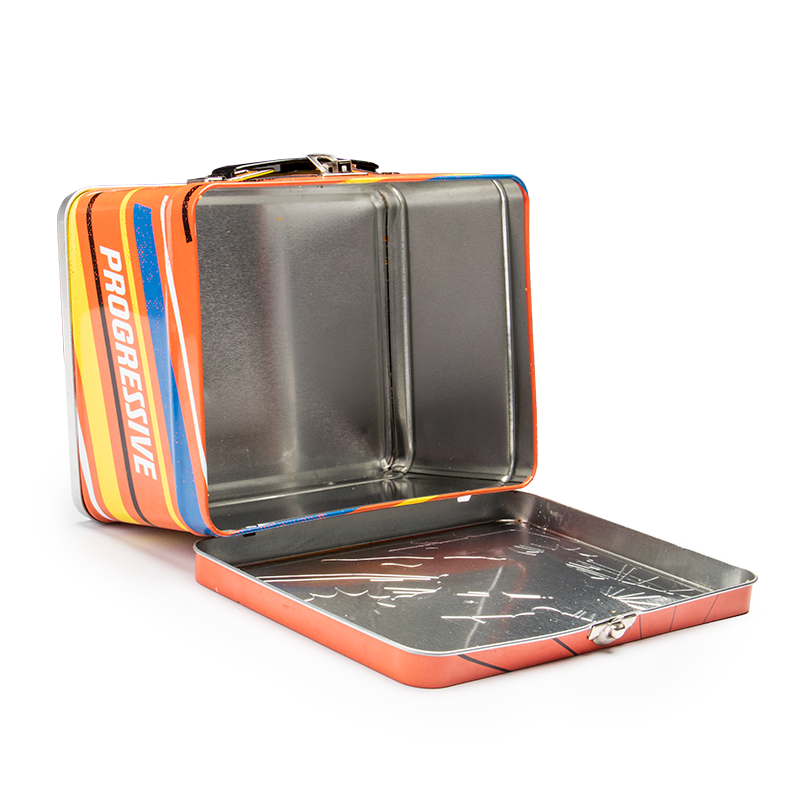This photograph depicts an open metal lunchbox, lying on its longer side against a stark white background, with the lid unlatched and lying flat, revealing the clean, shiny silver aluminum interior. The lunchbox features a bright, multi-colored exterior primarily dominated by orange, adorned with yellow, blue, and thin white stripes. Bold white lettering spells out "PROGRESSIVE," indicating a promotional item for the Progressive Insurance Company. The lid's rim matches the orange color of the box and contains some scratches. The lunchbox lacks a handle, emphasizing its possible multifunctional use.